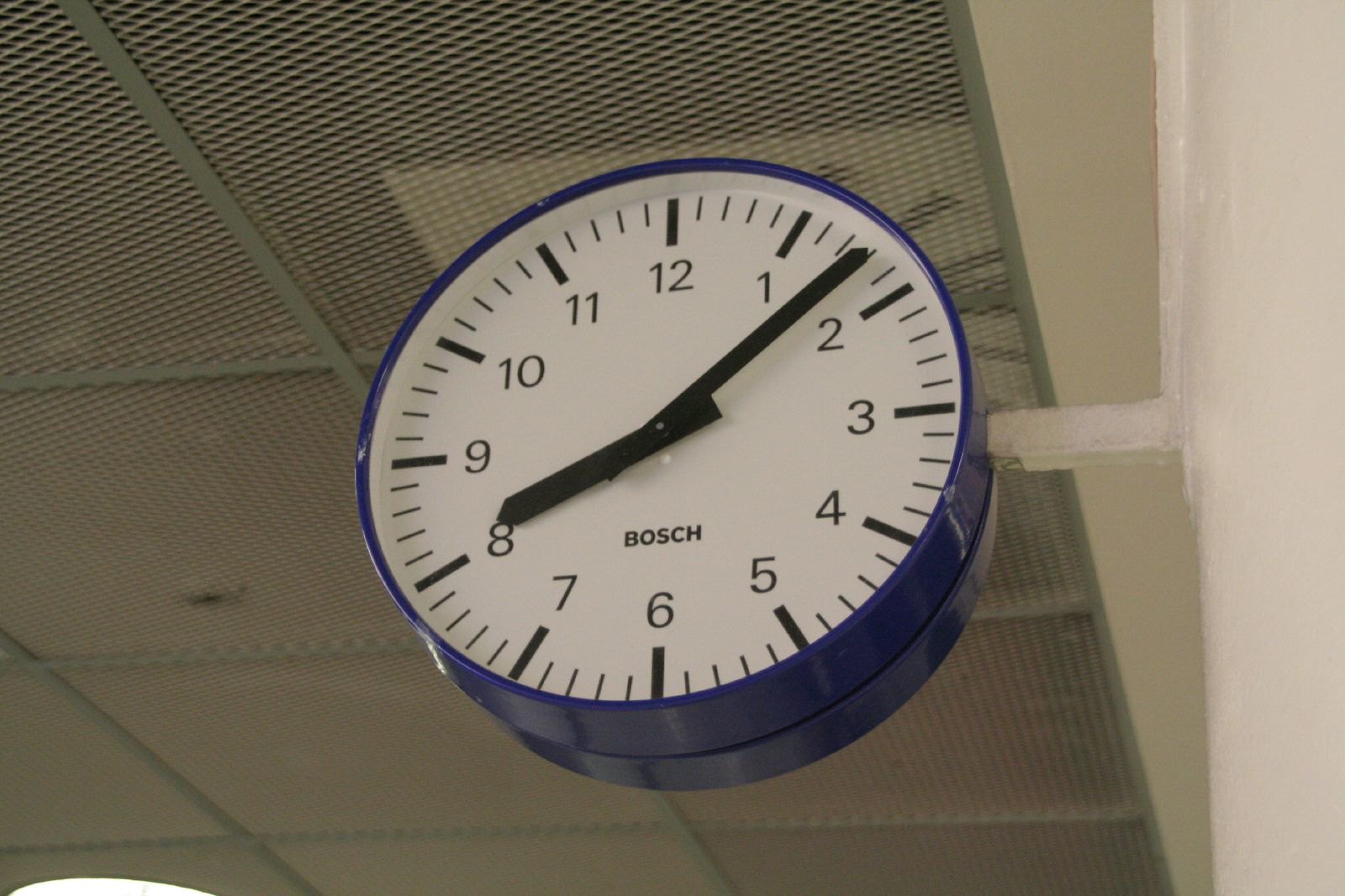The photo is a horizontal, full-color image capturing a clock affixed to a wall, viewed from below. The clock shows the time as 8:08 and features a simple, block-style numbering system from 1 to 12, in plain black font without any cursive or ornate details. The clock face is white, with each hour marked by a slightly darker black line, and additional ticks marking the minutes in between. Absent of a second hand, the clock has only black hour and minute hands. The clock's frame is a vibrant blue, contrasting starkly against the white wall. Above the clock, there is a mesh ceiling tile commonly found in office buildings, suggesting the location is likely an office environment. The brand "Bosch" is prominently displayed on the clock face.